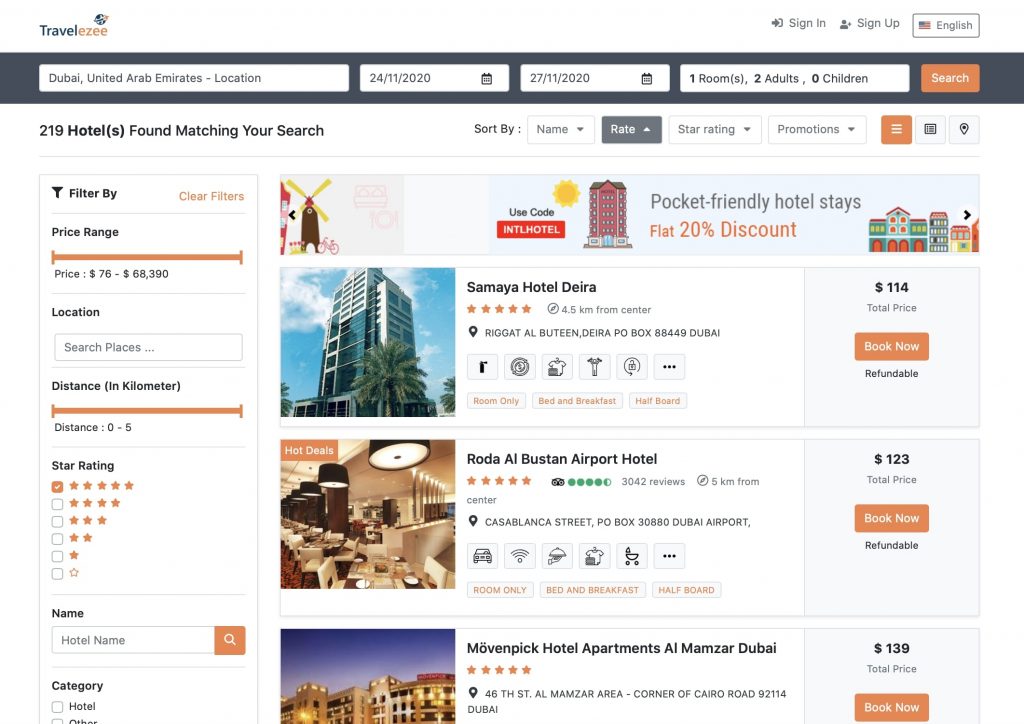**Image Description: Detailed Overview of a Travel Booking Website**

- **Header Section:**
  At the top left of the image, set against a mostly white background, the text "TRAVEL EASY" is prominently displayed. To the right of this text are several buttons, including a "Sign In" button, a "Sign Up" button, and a language selection button currently displaying "English." 

- **Search Bar:**
  Below the header, there's a dark bluish bar providing various search options:
  - The first text box displays the entry "DUBAI, United Arab Emirates" (location).
  - The next two boxes contain date selectors with the dates "24-11-2020" and "27-11-2020" respectively.
  - Following these is a box indicating "1 room, 2 adults, 0 children."
  - At the end of the bar is an orange search button.

- **Search Results Summary:**
  Beneath the search bar, there's a summary indicating that "219 hotels found matching your search" displayed on the left. To the right of this summary, there are various sorting options:
  - A "Sort by" dropdown.
  - A grey "Rate" button.
  - Dropdowns for star rating and promotions.
  - An orange calendar box with white icons, another location selector.

- **Filters:**
  On the left side of the screen, beneath this summary, there's a "Filter By" section including:
  - A "Clear Filter" option.
  - A price range slider.
  - A location search box.
  - A distance slider.
  - A star rating filter (0 to 5 stars).
  - A name entry box.
  - A category section which is partially cut off, only "hotel" is visible.

- **Advertisement Banner:**
  To the right of the filters, there is an advertisement banner reading "Pocket Friendly Hotel Stays" with illustrated hotel buildings. Below this, it reads "Flat 20% Discount" in orange text.

- **Hotel Listings:**
  Below the advertisement, there are several detailed hotel listings:
  - **Hotel 1: Semiya Hotel, Deira**
    - 5 stars, 4.5 KM from the center.
    - Address: Pin, Regat, Al Boutin, Deira, PO Box 88449 Dubai.
    - Icons representing amenities: spray bottle, coin, clothes, gym, lock, and three dots.
    - Tags: room only, bed and breakfast, half board.
    - Image: A large silver building.
    - Pricing: $114 total price, with a "Book Now" button.
    - Refundable option.

  - **Hotel 2: Rota Al Boutin Airport Hotel**
    - 5 stars, with an average of 4 stars from 3042 reviews, 5 KM from the center.
    - Address: Casablanca Street, PO Box 30880 Dubai Airport.
    - Icons: pin, car, Wi-Fi, lamp, clothes, baby bassinet, and three dots.
    - Tags: room only, bed and breakfast, half board.
    - Image: Fancy dining room.
    - Pricing: $123 total price, with a "Book Now" button.
    - Refundable option.

  - **Hotel 3: Movenpick Hotel Apartments Al Mamsar Dubai**
    - 5 stars.
    - Address: 46th Street, Al Mamsar area, corner of Cairo Road, 92114 Dubai.
    - Image: Blue sky with a set of buildings.
    - Pricing: $139 total price, with a "Book Now" button.